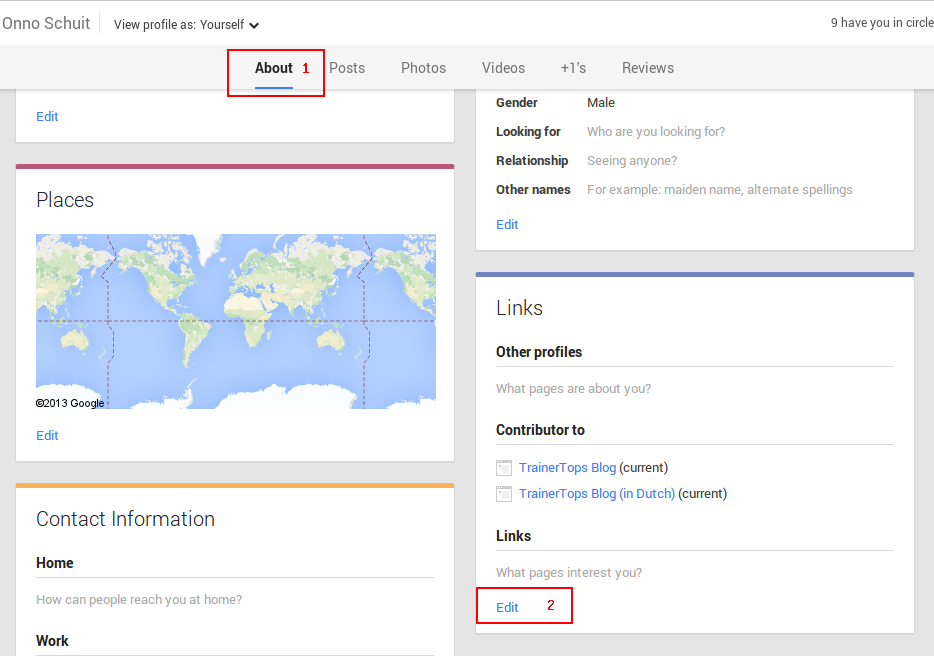This image depicts a screenshot of a user profile page, most likely from a social media platform. At the very top of the screen, there's a heading with the text "Oh No Schuit," written as "O-N-N-O S-C-H-U-I-T." Just beneath this heading, there's an option labeled "View profile as yourself."

Centered below this option is a navigation menu featuring the headings: "About," "Posts," "Photos," "Videos," "Plus Ones," and "Reviews."

On the left side of the screen, there is a section titled "Places." This section displays a Google map showcasing the continents and predominantly features a lot of blue regions, indicating water bodies such as oceans and seas.

Below the map, another box is labeled "Contact Information." Within this section, two categories are shown in bold: "Home" and "Work." "Home" is followed by the prompt "How can people reach you at home?" which is written in gray text. The "Work" section does not have any additional text displayed.

On the right side of the screen, starting from the center, there's a box containing several personal details: "Gender: Male," "Looking for: Who are you looking for?", "Relationship: Seeing anyone?", and "Other Names: For example, maiden name, alternate spellings."

The detailed layout and headings form a comprehensive user profile, combining contact information, personal details, and navigation options.